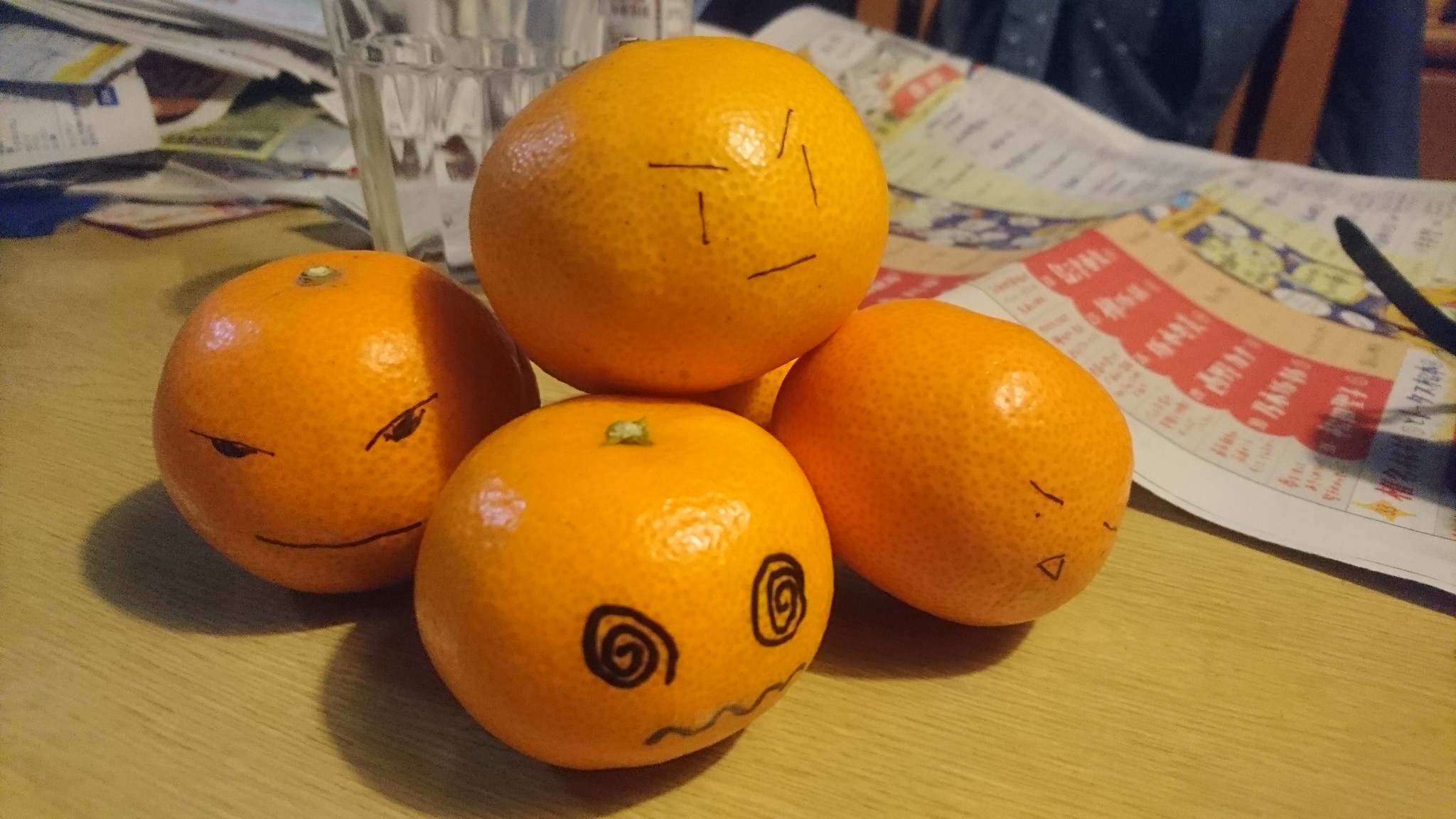This color photograph depicts an organized yet lively desk scene, centered around five oranges methodically stacked atop a light-colored wooden table. Each orange has a whimsical face drawn on it with a marker, resembling Halloween jack-o'-lanterns. Starting with the facial details, one orange features angry eyes and raised eyebrows conveying a solemn look. Another is marked with swirly eyes and a wavy mouth, suggesting confusion or dizziness. A third sports a triangle nose and appears happy despite lacking a mouth. The fourth has simple vertical lines for eyes, a straight line for a mouth, and expressive eyebrows hinting at frustration. The final orange has slitted eyes and no mouth, possibly portraying sleepiness.

Nestled among the oranges is a see-through glass, half full of water. In the background, a neatly spread out newspaper occupies the desk, along with other indistinguishable papers in the left-hand corner, possibly unopened mail. The scene merges everyday life with a touch of creative whimsy.